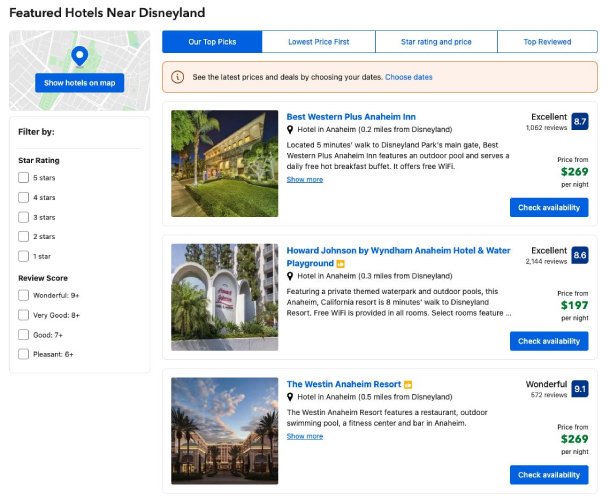The screenshot captures a webpage listing hotels near Disneyland, prominently indicated by the text "Hotels near Disneyland" at the top left. Below this header, a rectangular map section features a blue pin labeled "Show hotels on map" for geographic reference. Adjacent to the map on the right, there is a navigational bar with clickable options, currently highlighting "Our Top Picks" in blue. Additional sorting options, such as "Lowest Price First," "Star Rating and Price," and "Top Reviewed," are available along the same bar.

The webpage showcases three hotel options. The first entry is the Best Western Plus Anaheim Inn, accompanied by a thumbnail image. This hotel is rated 8.7, labeled "Excellent," with a nightly price of $269. A blue "Check Availability" button is available for reservation inquiries.

The second listing is the Howard Johnson by Wyndham Anaheim Hotel and Water Playground, rated 8.6, priced at $197 per night, also featuring a "Check Availability" button.

The final hotel is The Westin Anaheim Resort, depicted with an inviting image of palm trees and a blue sky sprinkled with clouds. This hotel boasts a rating of 9.1, described as "Wonderful," with prices starting at $269 per night. It too includes a "Check Availability" button for reservations.